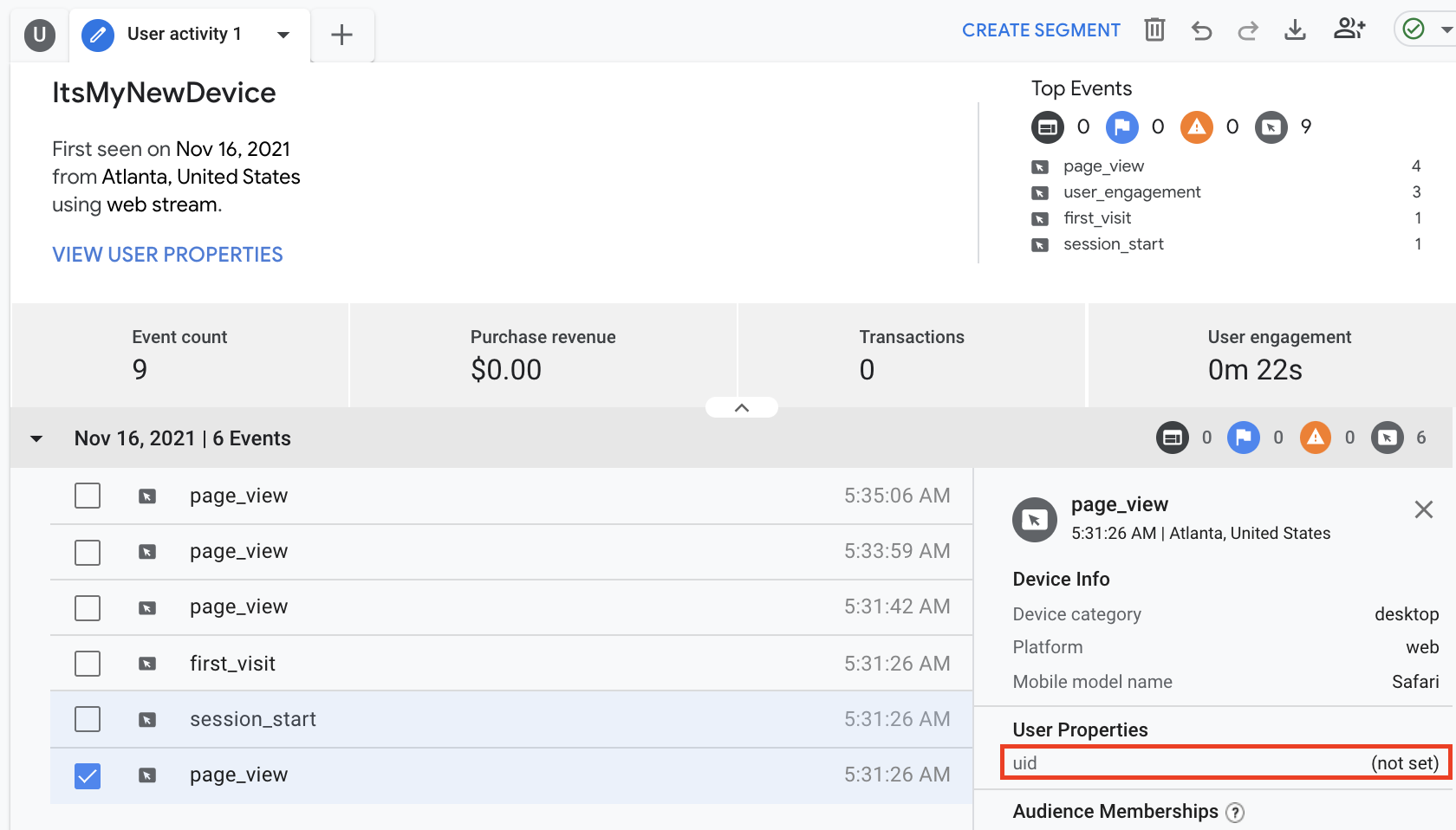This image depicts a webpage, possibly from a website or an application interface, featuring a detailed toolbar at the top. Starting from the left, the toolbar includes the following elements: a black circle icon with the letter 'U' in white font, a blue circle icon resembling a pen, and a tab labeled 'User Activity 1' in black font with a dropdown arrow. Adjacent to these is a plus symbol (+), followed by a series of functions on the right side: 'Create Segment' in blue font, a trash bin icon (delete feature), back and forward arrows, a download button, and a profile button. On the far right, there's a circle with a check mark and a dropdown arrow. All these elements are set against a greyish background. The currently active tab, 'User Activity 1,' is highlighted in white. Beneath this toolbar is a second row displaying the bold, larger text: "It's my new device."